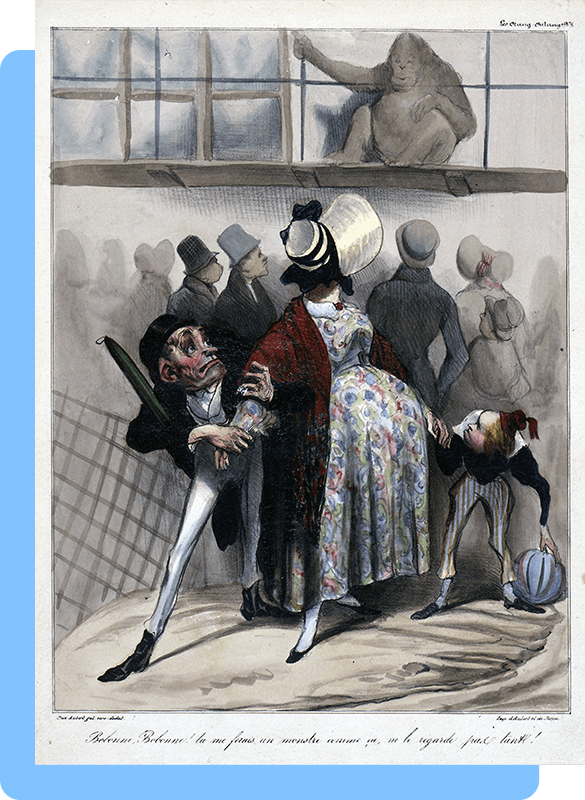The image depicts an intricately detailed, colored sketch resembling a caricature or political cartoon set within a square frame, bordered on the left and bottom by a light blue edge. At the top of the scene, a gorilla or orangutan sits on a platform, grasping a metal bar while looking down at a crowd of spectators below, who appear to be dressed in old-timey clothes. Among them is a prominently pregnant woman in the foreground, wearing a large white bonnet with a black ribbon, a floral dress in shades of blue, green, and red, and a red shawl. She faces the gorilla with her back to the viewer, exposing her large belly as she is gently pulled by a worried-looking man clutching her right arm. To her left, a shorter man with a small red cap and tassel holds her left hand and a ball. The lower part of the image contains black script text, possibly in a different language, which is difficult to decipher.